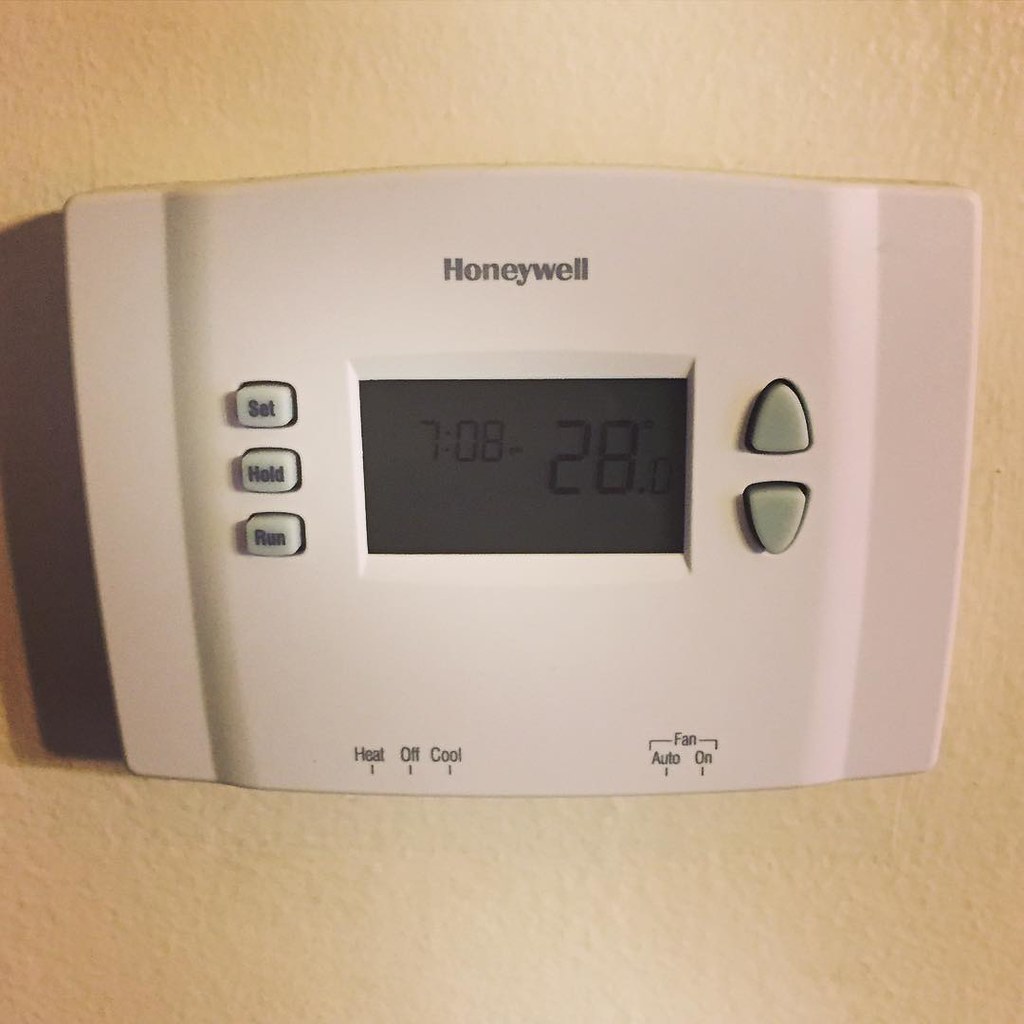The image depicts a white Honeywell thermostat mounted on a plain white wall. The thermostat is square in shape with a slightly protruding frame. On its left side, there are three white buttons labeled in black as follows: "Set," "Hold," and "Run" from top to bottom. Below these buttons, another set of labels read "Heat," "Off," and "Cool," as well as "Fan," "Auto," and "On." Each of these settings is accompanied by a black line that links to the corresponding labels.

The central display screen of the thermostat is not backlit but clearly shows the time as 7:08 and the temperature as 28 degrees Celsius. There is a pair of white buttons beneath the screen for adjusting the temperature up and down. The brand name "Honeywell" is printed in black near the top of the device.

Despite the lack of illumination, all the features of the thermostat, including the time, temperature, and various settings, are easily legible. The unit is securely affixed to the wall, with a slight lip giving it a three-dimensional aspect.